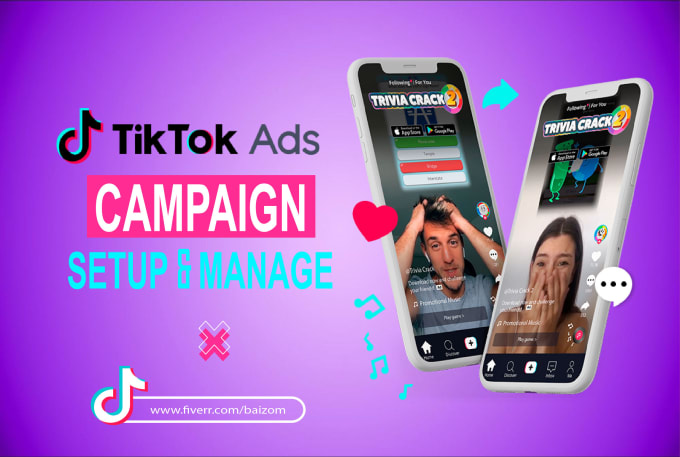The image features a vibrant purple background that transitions from dark at the edges and corners to a lighter shade at the center. Diagonally positioned in the middle are two smartphones displaying the game "Trivia Crack 2" at the top of their screens. 

The phone on the left shows a young, fair-skinned man with tousled hair, who appears to be experiencing amused frustration. On the right phone, a young, fair-skinned woman with dark hair is captured mid-laugh, her mouth covered with both hands in a gesture of amusement. 

To the left of the leftmost phone is a TikTok music note icon followed by the text "TikTok Ads Campaign Setup and Manage." Below this is the TikTok logo and a URL: "www.fiverr.com/baizom." Scattered around the left phone are several floating turquoise music notes and a red heart icon, enhancing the playful theme of the image.

On the right side of the rightmost phone is a white text bubble with three horizontal black dots, indicating an ongoing communication or typing indicator, adding an interactive feel to the scene.